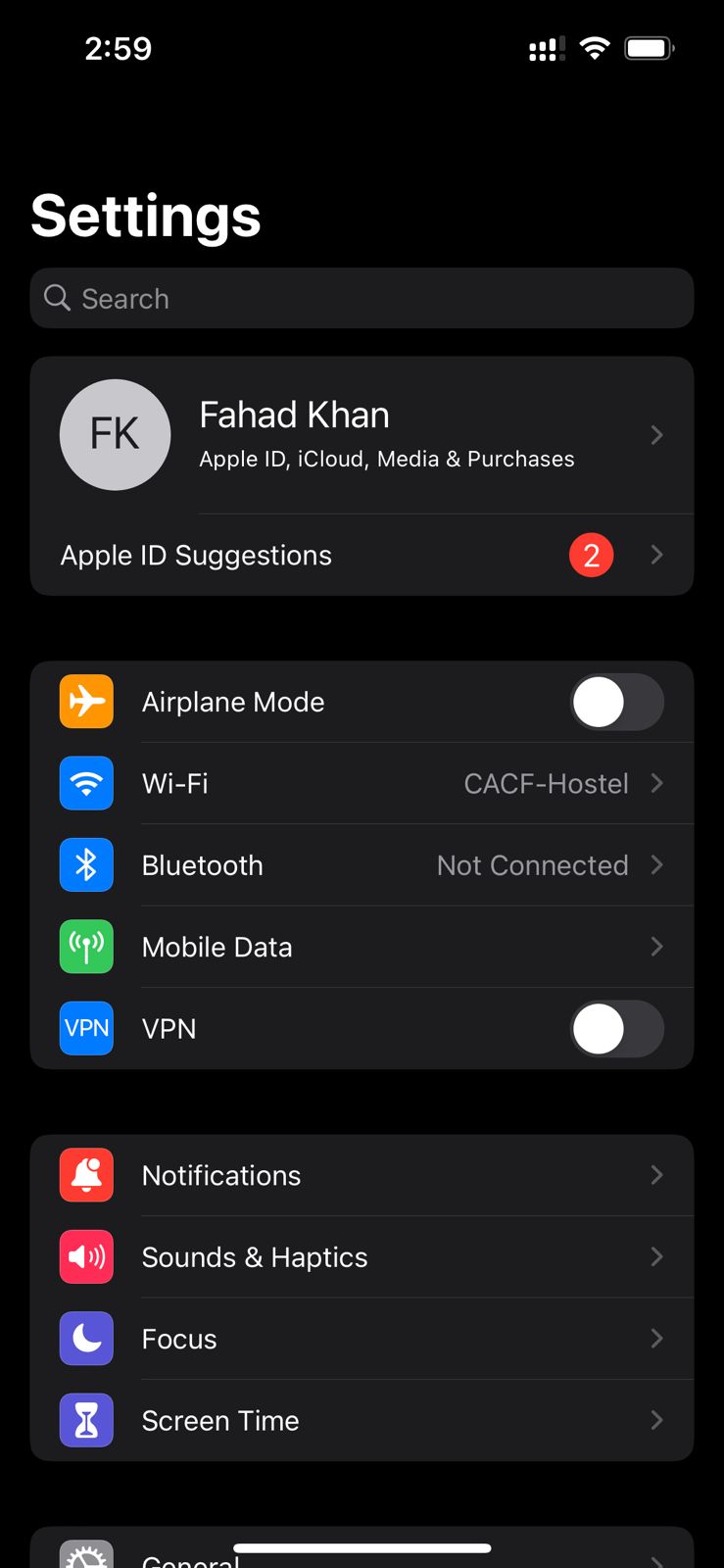This is a detailed screenshot of a cell phone displaying the "Settings" menu. The background of the screenshot is black. At the top left corner, the time is shown in white text. On the top right corner, there are icons for reception, Wi-Fi, and battery status. 

About five lines down from the top, there is a large, bolded white heading that says "Settings". Below this heading is a grey search bar with a magnifying glass icon and the word "Search" in grey on the left-hand side.

Moving further down, there is a black rectangle. In the upper-left corner of this rectangle, there is a light grey circle containing the black capital letters "FK". To the right of this circle, the person's name is displayed. Directly below the name, in white text, it says "Apple ID Suggestions". On the right side of this section, there is a red circle with a white number "2" inside it, indicating notifications. Both lines have a right-pointing grey arrow that looks like a sideways "V".

Following this section, there are two menu options, each situated within its own rectangle and accompanied by icons to the left. The first option is "Airplane Mode" with a toggle switch to the right. The second option is "Wi-Fi" with the text "CACF-hostile" in grey to the right and a right-pointing grey arrow.

Below these, there are more settings options listed in rectangles:
- "Bluetooth" which indicates "Not Connected" on the right and a grey arrow.
- "Mobile Data" followed by a grey arrow.
- "VPN" with a toggle switch to the right.

After a small black space, another segment of menu options appears, each within its own rectangle and accompanied by icons:
- "Notifications"
- "Sounds & Haptics"
- "Focus"
- "Screen Time"

Each of these options has a right-pointing grey arrow that looks like a sideways "V". At the very bottom of the image, the top portion of another rectangle is partially visible.